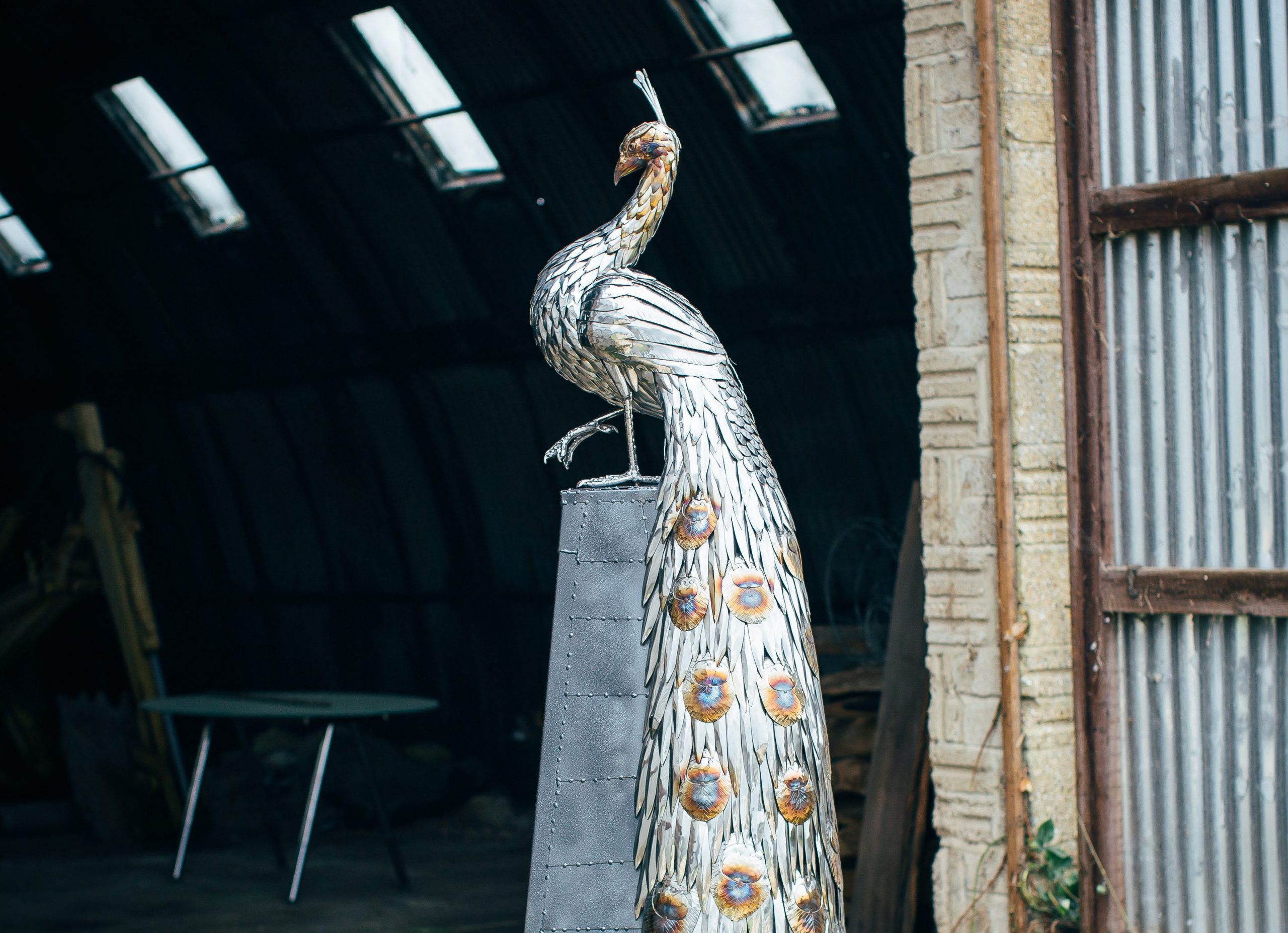The image depicts a detailed statue of a white peacock with a side profile, its plumes laying flat and adorned with colorful spots in shades of brown, blue, and gray, giving the impression of brass and blue hues. The peacock stands majestically atop a tall metal stand, situated at the edge of what appears to be a dimly lit warehouse or garage. The background features a dark space with some light streaming in from four slanted windows. The left side of the image is predominantly dark, revealing only a hint of the interior, while the right side shows a gray wall accompanied by steel plates, rusty steel boards, and a brick face with a light brown hue. Additionally, a green tabletop with silver legs and a brown metal pole can be seen within the space, adding to the eclectic environment surrounding the statue.